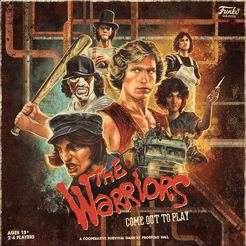This is a detailed color movie poster for the film "The Warriors." The central portion of the poster is populated with several characters from the movie, arranged one in front of the other. In the foreground on the left, there's a man dressed as a baseball player, complete with a black hat and makeup, and he is holding a baseball bat, ready to swing. Next to him, there is another man wearing a blue hat who appears to be shouting angrily. In the center, a blond man with short hair and a red vest stands prominently. To his right, a woman holds a knife menacingly. 

Additionally, on the right side of the poster, there is an image of a van with people both inside and on top of it. The background features a network of sewer pipes against a black backdrop, adding to the gritty urban atmosphere. At the bottom of the poster, bold red text declares the film's title, "The Warriors," with the white subtext "Come Out To Play" beneath it. There is also smaller white text at the bottom, though it is not legible.